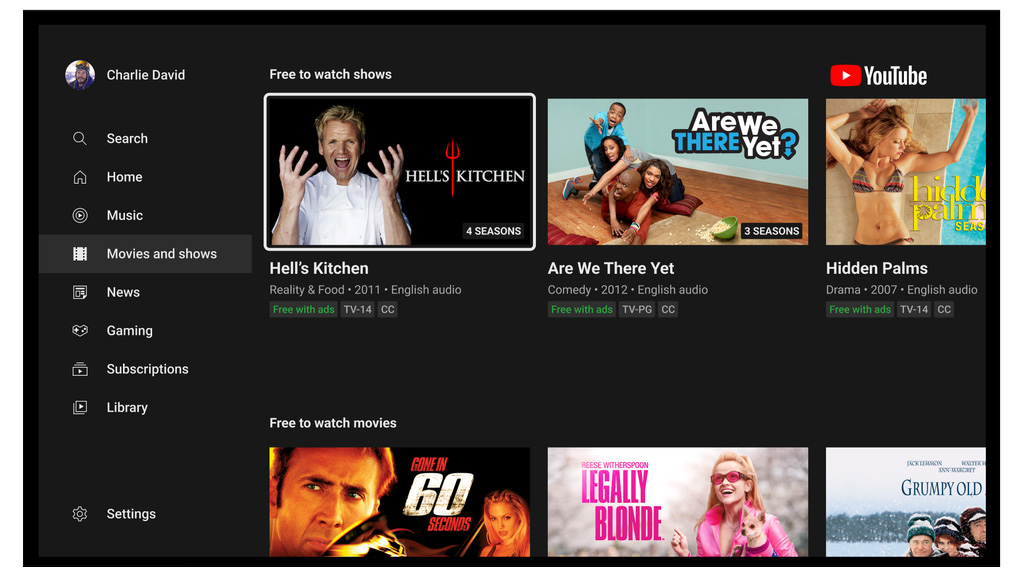This is a detailed screenshot of a Spotify interface showcasing a user's account and the Movies and Shows section. The overall background is black, providing a sleek and immersive visual experience. On the left side, there's a sidebar containing user information. At the very top of the sidebar, a profile picture and the name "Charlie David" are displayed prominently. Below this, a list of Spotify's navigation options is presented, each accompanied by an icon to the left. 

The navigation buttons in order are:
1. Search
2. Home
3. Music
4. Movies and Shows
5. News
6. Gaming
7. Subscriptions
8. Library

A considerable gap follows these, and the "Settings" button is located at the very bottom of the sidebar.

Moving to the main content area, the "Movies and Shows" section is in focus. At the top of this section, the heading "Free to Watch" is displayed. Below the heading, there are six featured videos arranged in two rows. 

In the first row of videos:
1. "Hell's Kitchen" (2011) – This video is tagged "Free with ads" in green and has a TV-14 rating.
2. "Are We There Yet?" (2012) – This video also has a "Free with ads" tag.
3. A YouTube video titled "Hidden Palms" (2007) – Also marked "Free with ads".

In the second row of movies below:
1. "Gone in 60 Seconds"
2. "Legally Blonde" in the middle
3. "Grumpy Old Men" on the far right

The screenshot effectively captures the diversity and accessibility of content available on Spotify’s Movies and Shows section, emphasizing user-friendly navigation and a rich selection of ad-supported free content.